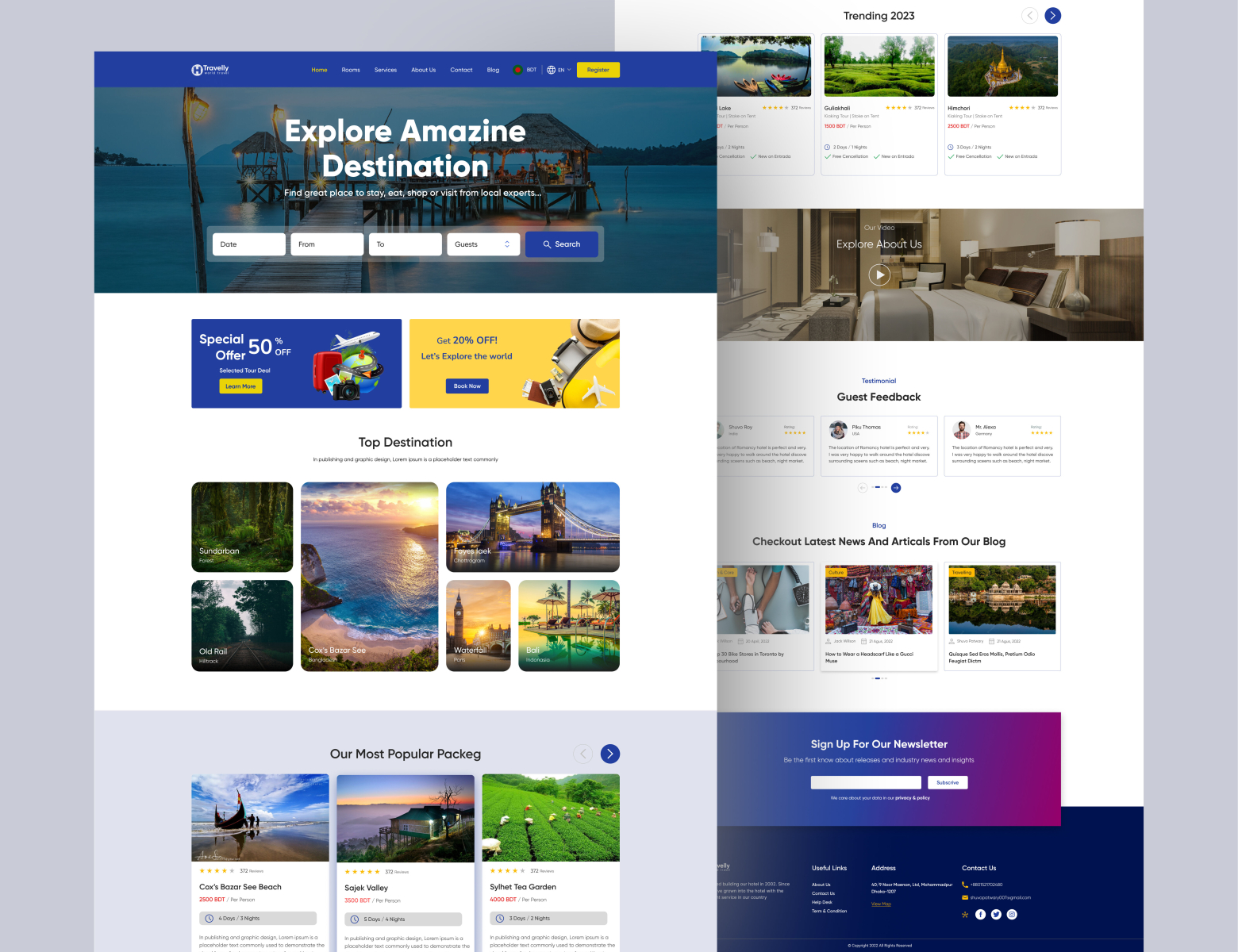The image showcases a layered view of two web pages. The page on the left overlaps the left portion of the page on the right. The left page features a blue bar running across the top with various menu options. Below this bar, there is an image of a serene waterfront setting, complete with a dock leading to small wooden huts, accompanied by the text "Explore Amazing Destinations." Following this image, there are four search fields arranged horizontally, ending with a blue search button. Beneath the search section, set against a white background, is a prominent special offer announcing "50% off", alongside a smaller yellow square marketing a "20% off" discount. This section is followed by two distinct groups of images showcasing various attractive destinations to explore.

The right page is organized with three destination photographs displayed across the top. Below these images, an expansive picture depicts the interior of a hotel room, complete with a comfortable bed, three lamps, and a brown door. Further down, the page headline "Check Out the Latest News and Articles from Our Blog" introduces another set of three images. At the very bottom, there is a call to action inviting visitors to sign up for the newsletter.